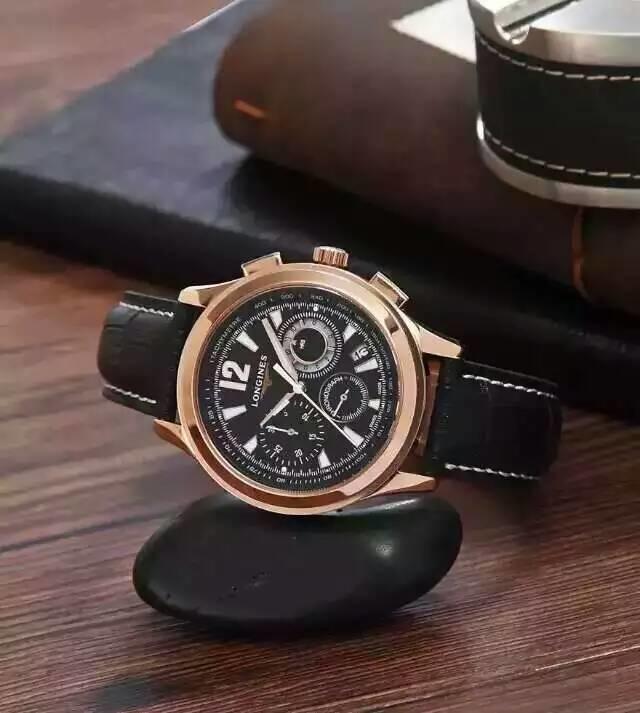This photograph showcases a detailed watch displayed on a dark brown wooden table with black grain spots. The watch rests on a black, egg-shaped support, possibly a polished rock or charger, which has an indent to fit the watch. The timepiece features a gold bezel and a black dial with white markings. The band is crafted from black leather with white stitching along its edges. The watch face includes the number 12 at the top and various smaller dials with intricate details indicating barometric pressure and possibly a compass. The time shown is approximately 10:08, with the second hand at the 36-second mark. Surrounding the main dial are additional round dials located at the 3, 6, and 9 o'clock positions. In the backdrop, there are leather-bound books in black and brown, adding a scholarly essence to the composition.